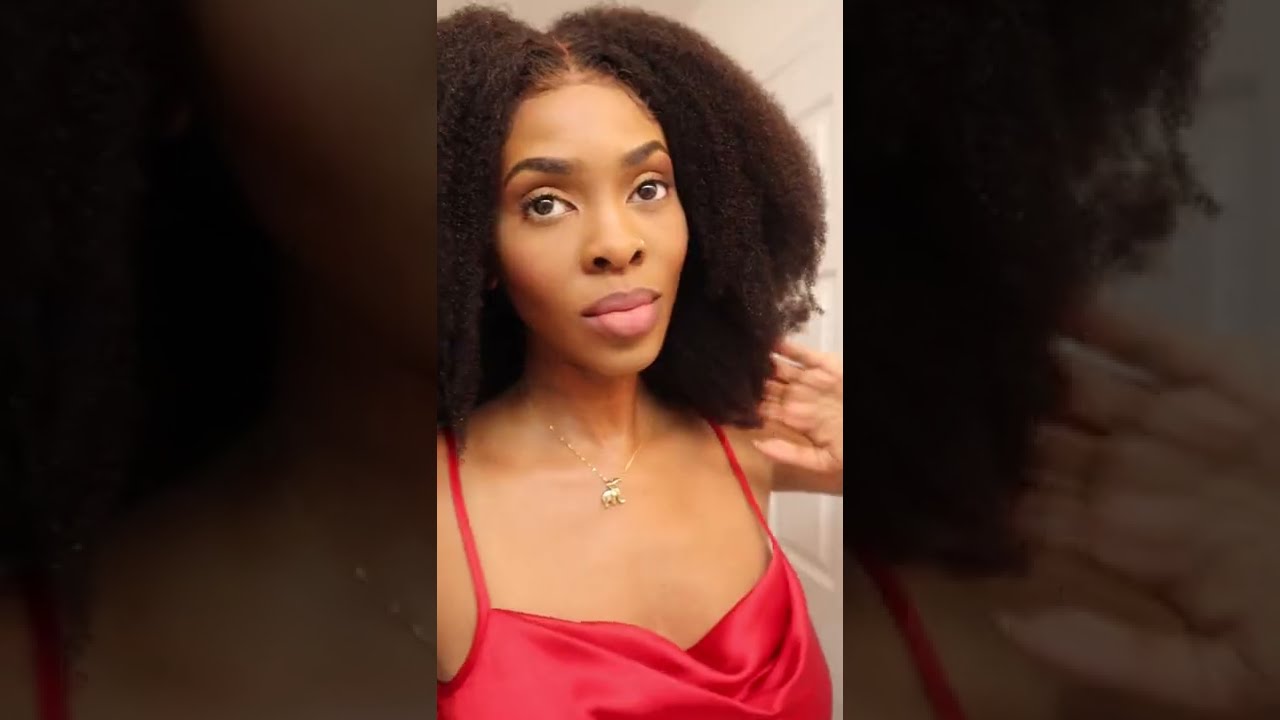The photograph features an African-American woman with a deep brown complexion and long, frizzy, dark brown to black hair parted at the center that falls down to her shoulders. She is taking a selfie, evidenced by the vertical crop typical of phone photos. The woman has soft brown eyes and full, pinkish lips, with a slight smile as she looks up into the camera. Her head is gently tilted to the left, and she appears to be in her late 20s.

She’s adorned with a golden necklace, featuring a small, gold ornament that resembles an elephant. The woman is wearing a bright red, velvety teddy or camisole that exposes her shoulders and has thin straps. The top is satiny and loose-fitting, highlighting her chest area. Her left hand is raised near her hair, revealing the palm side.

The background is mostly shadowy, with a blown-up, more shadowy version of the same image providing a layered effect. A sliver of white wall and possibly a white door can be seen behind her, contributing a subtle contrast to the photograph’s composition.